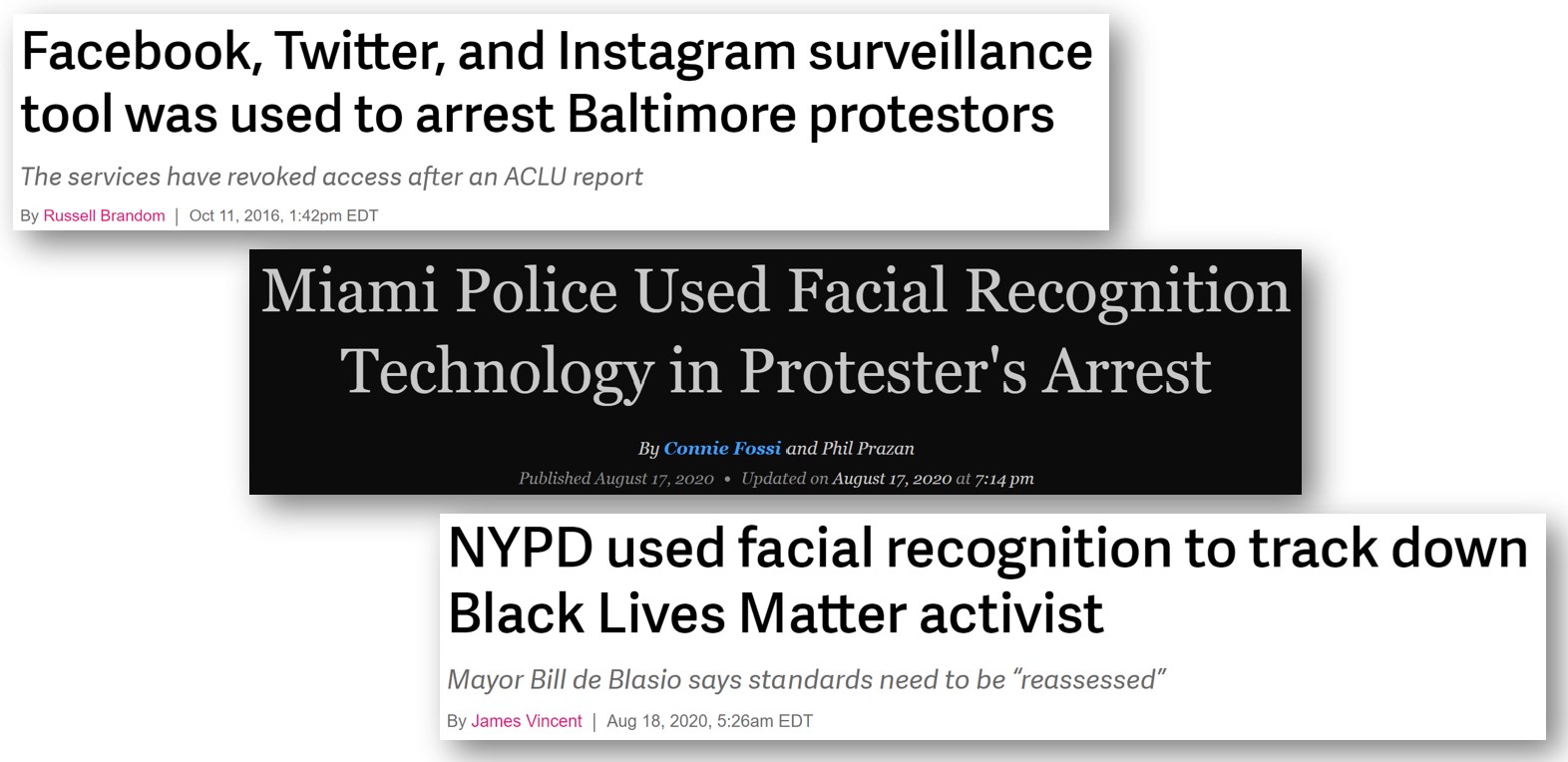Screenshot showing three different articles highlighting the controversial use of surveillance and facial recognition technology by police on protesters:

1. The first article features the title: "Facebook, Twitter, and Instagram Surveillance Tool was Used to Arrest Baltimore Protesters." Introductory text below the title states that these services revoked access after an ACLU report.
   
2. The second article titled "Miami Police Used Facial Recognition Technology in Protester's Arrest," set against a stark black background.

3. The third article, on a white background, is titled "NYPD Used Facial Recognition to Track Down Black Lives Matter Activists." Beneath the title, it notes Mayor Bill de Blasio's call for a reassessment of scanners.